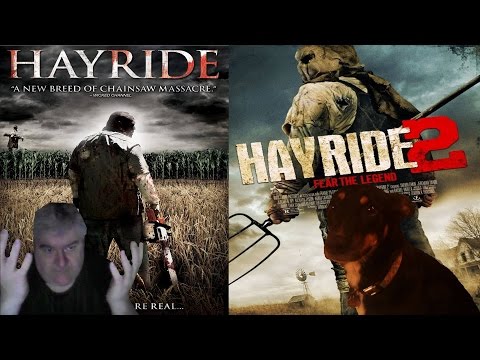This small, horizontally aligned rectangular image is bordered by thick black bars at the top and bottom, framing two movie cover posters side by side. The left poster is for "Hayride" with the tagline, "A New Breed of Chainsaw Massacre." It depicts a spooky scene with a field of tall corn and dead weeds, where a scarecrow stands and a man in dark, ragged clothing with a chainsaw in his right hand walks away from the viewer. In the lower left corner, there is an image of a man with short black and gray hair, light skin, and a dark shirt, his hands raised in a defensive gesture, accompanied by the text "Be Real" in the lower right corner.

The right poster is for "Hayride 2" with the tagline, "Fear the Legend" in red text beneath the title. This cover features a man in similar ragged clothing, shown partially from behind, holding a pitchfork. He wears a mask, and a dog with a collar sits in front of him, staring directly at the camera. The overall style of the image gives a poster-like appearance, combining spooky rural elements and ominous figures, enhancing the horror theme of both movies.